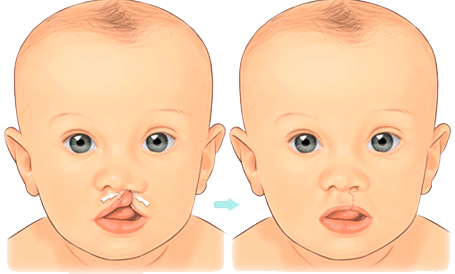This is an illustration depicting a detailed before-and-after comparison of a baby who underwent surgery for a cleft lip. Set against a plain white background, the rectangular artwork measures approximately three inches wide by two inches high. The drawings, which show the baby from the shoulders up, portray an infant with light skin and a wisp of brown hair. The baby’s gray-blue eyes are prominent in both images. 

On the left half of the drawing, the baby is depicted with a cleft lip, where the top lip is connected to one of the nostrils, causing the right nostril to appear slanted. The image includes two white arrows pointing to the cleft lip to highlight the condition. On the right side, the same baby is shown post-surgery with a repaired lip that forms a regular bow shape and a subtle scar running from the lip to the nostril. A blue arrow points from the "before" image on the left to the "after" image on the right, effectively contrasting the baby’s appearance before and after the surgical correction.